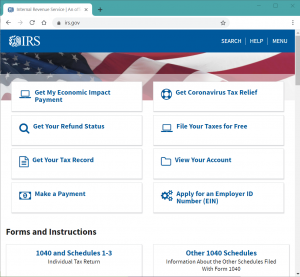The website for the IRS at irs.gov features a blue navigation bar at the top. On the left side of this bar, the letters "IRS" are prominently displayed in capital letters. To the right, the options "Search," "Help," and "Menu" are listed. Below the navigation bar, a partial image of the United States flag is visible, showcasing some stars along with the red and white stripes.

Beneath the flag, the content is organized into two vertical columns. The left column, from top to bottom, includes the following blue links accompanied by icons:
1. Get My Economic Impact Payment
2. Get Your Refund Status
3. Get Your Tax Record
4. Make a Payment

The right column, also featuring blue links with icons, lists:
1. Get Coronavirus Tax Relief
2. File Your Taxes for Free
3. View Your Account
4. Apply for an Employer ID Number (EIN)

Below both columns, the phrase "Forms and Instructions" appears in black text.